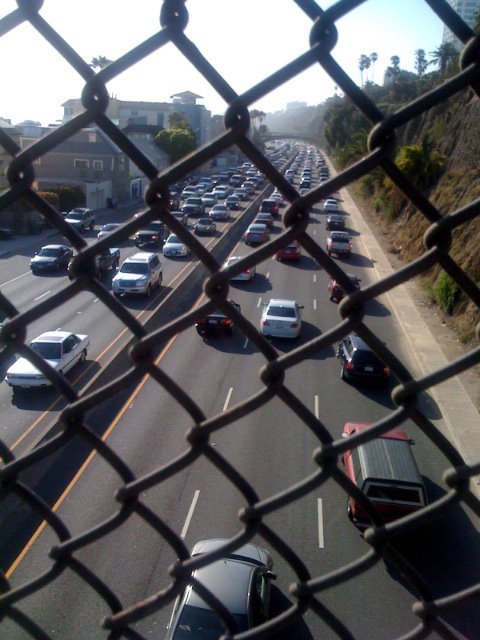The photograph captures a bustling highway, viewed from a pedestrian overpass through a black chain-link fence. The image reveals six lanes of traffic, three in each direction, separated by a concrete divider. Yellow lines mark the outer edges of the road, while dotted white lines distinguish the lanes. The roadway is flanked by two contrasting landscapes: to the right, a steep hill adorned with green vegetation and some trees, including palm trees, peaks with a building perched atop; to the left, a residential area featuring houses and additional trees. The scene is bathed in sunlight under a grayish-blue sky, suggesting a hot, clear day. The traffic appears dense, extending uninterrupted down the highway in both directions, indicating a busy thoroughfare.